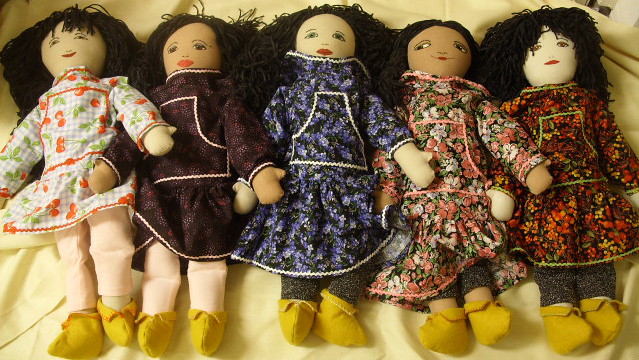This image captures five diverse cloth dolls lying on a cream-colored blanket. Each doll, approximately 18 inches to 2 feet tall, features long black yarn hair and distinct facial details, including red lips and small cloth eyes. They have various skin tones ranging from very fair to very dark, highlighting their diversity. 

The dolls are dressed in an array of patterned outfits, with three wearing flower dresses in different colors, one in a plain brown dress with white piping resembling leather, and the last in a gingham dress. Despite the variety in their clothing, the dress shapes are similar. Additionally, they all wear different colored tights and yellow shoes, often described as moccasins. 

Each doll lies flat on its back with its arms crossed over the adjacent doll, creating a harmonious arrangement. The dolls' hands are simple, lacking fingers, and are made entirely of cloth. The photograph emphasizes the uniqueness and diversity of each doll while maintaining a sense of unity in their arrangement and styling.